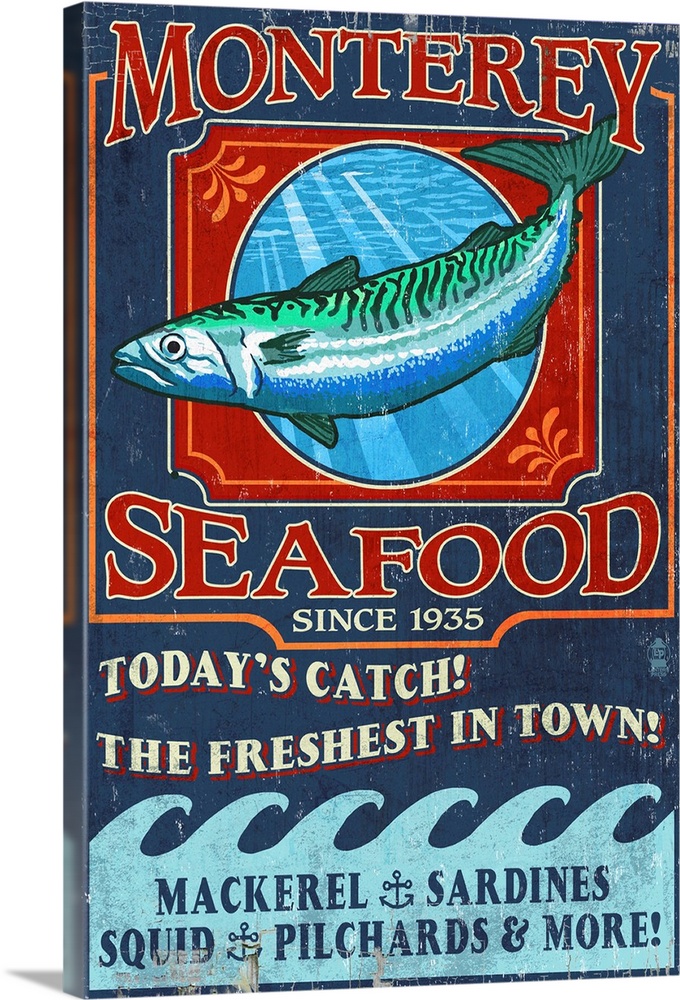This is a photo of a vintage-style advertisement for Monterey Seafood, likely intended to be hung on a wall. The ad, which has a weathered and aged appearance with visible smudges and chunks missing, features a prominent image of a large painted fish with green fins, a silver center, a bright green top with black stripes, and a white eye with a black center. The fish appears within a blue circle with sun rays penetrating the water and is framd by a red trim with a leaf design in the corners. 

At the top of the ad, "Monterey Seafood" is written in red block letters, with "Seafood" and "Since 1935" written underneath in white text. Beneath this, the text reads, "Today's catch, the freshest in town!" also in white with a slight red shadow. The bottom portion features light blue painted waves, with the names of various seafood—mackerel, sardines, squid, pilchards, and more—listed in darker blue text on top of the waves. The sign has a vintage, thick canvas-like appearance, contributing to its aged charm.